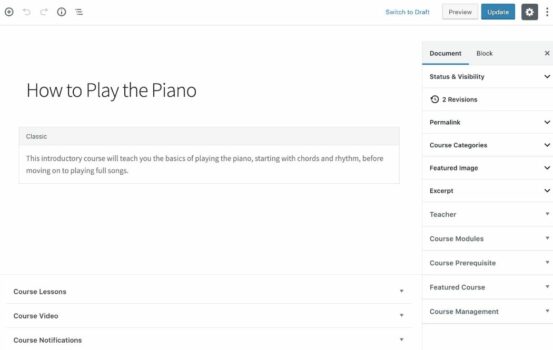The image is a screenshot of a web page open on a computer, featuring an introductory course titled "How to Play the Piano." Centrally located, the title is prominently displayed, followed by a description that outlines the course's content. This course promises to teach the basics of piano playing, beginning with chords and rhythms, and progressing to entire songs.

In the bottom left-hand corner, there are three clickable links for "Lessons," "Course Video," and "Course Notifications," providing users with various resources to enhance their learning experience. To the right, there is an extensive list of documents available for viewing and clicking, ensuring comprehensive coverage of the subject matter.

At the top right-hand corner, users can find a "Preview" button and an "Update" button, accompanied by a settings icon, allowing for easy navigation and customization of the course interface. The interface features a clean, white background, contributing to its straightforward and user-friendly design.

On the top left-hand corner, a back button and a forward button facilitate seamless browsing through the course materials. This web page appears to be a dedicated portal for an educational tutorial on piano playing, offering multiple courses, instructional videos, and lesson notifications. The title "How to Play the Piano" is prominently displayed towards the left center of the page, emphasizing the primary focus of the content.